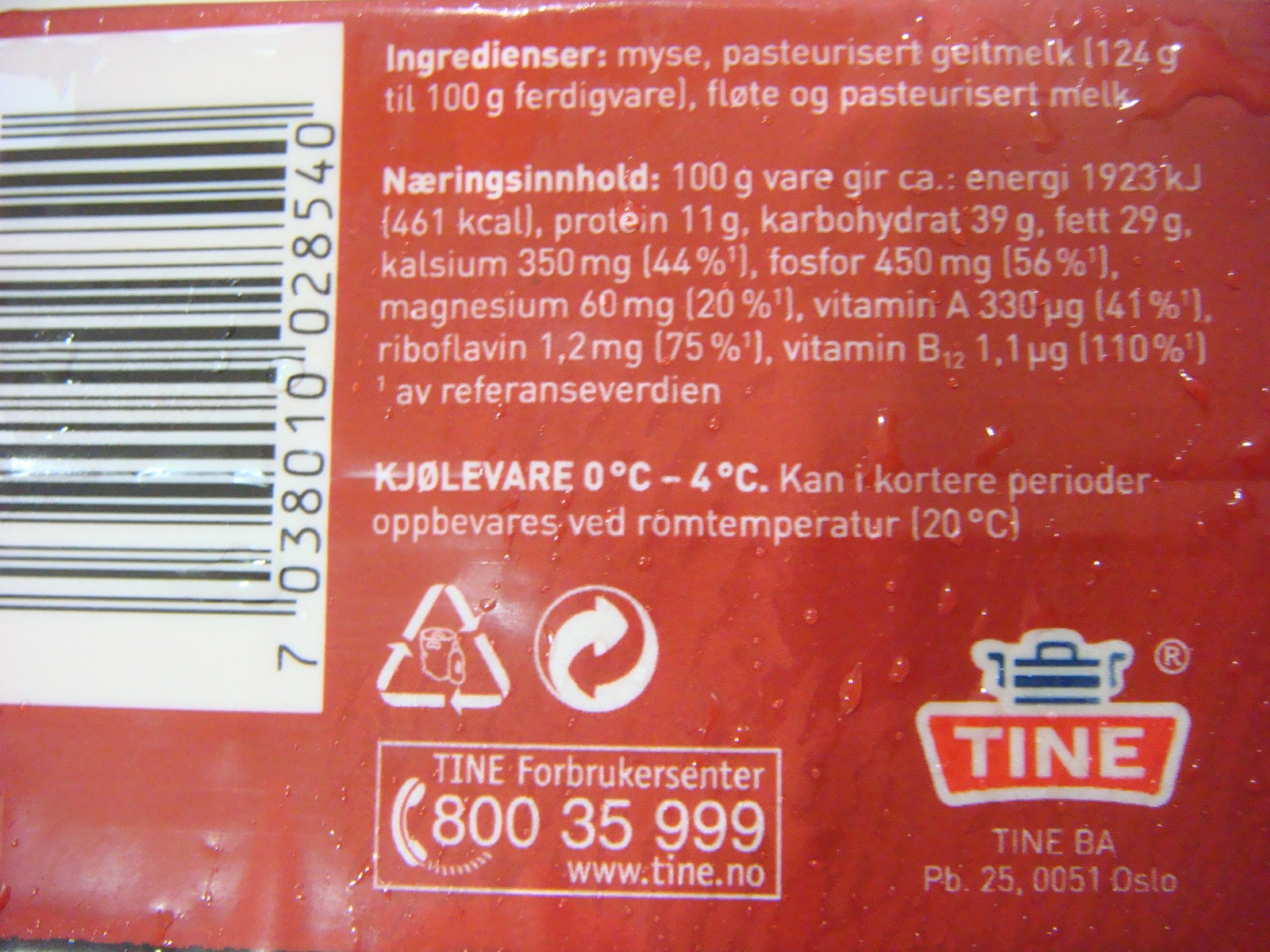The image shows the back of a red food packaging, featuring labels and details written in white text. The packaging appears to be in a non-English language with some similarities to English. A white rectangular area in the left-hand corner contains a black barcode with the number 7038010028540 printed in black. Above the barcode, bolded titles like "INGREDIENSER" and "NAERINGSINNHOLD" are followed by lists of ingredients and nutritional information, including "vitamin A-330" with an unidentifiable unit of measure. The label also consists of smaller symbols often used in food packaging, including recycling details and a blue pot symbol with two handles. Additionally, there's a logo spelling "TINE" inside a white shape, indicating the product is connected to or manufactured by TINE, likely in Oslo as suggested by the lettering beneath. The red background features water droplets, adding texture to the packaging.